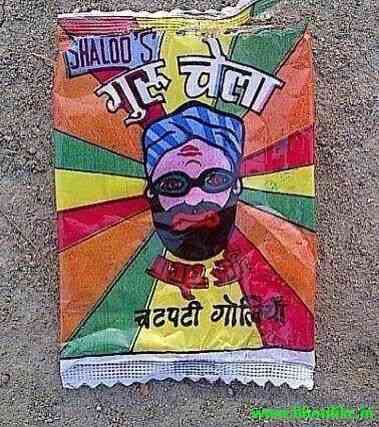This photograph, likely taken outdoors, features a low-resolution and heavily compressed image of a ripped open candy wrapper resting on what appears to be gray concrete. The rectangular wrapper is adorned with vibrant stripes of orange, green, yellow, and red radiating from its center. Dominating the middle of the wrapper is a cartoon-like face of a bearded man with red lipstick, wearing black goggles and a blue striped turban. The text "Shall Lose" is prominently displayed in the top left corner, set against a blue box, while additional text, possibly in Arabic, is positioned above and below the illustrated face. The lower right corner contains some illegible text due to the image's poor quality.